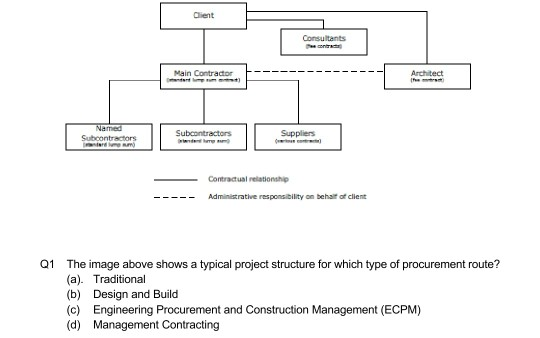The image displays a detailed flowchart against a white background, illustrating a typical project structure. At the top center, a box labeled "Client" is positioned, with a box labeled "Consultants" to its right and "Architect" to the right of the Consultants. Directly below the Client box is another box labeled "Main Contractor." From the Main Contractor, three boxes extend downwards, labeled "Named Subcontractors" on the left, "Subcontractors" in the middle, and "Suppliers" on the right. 

Arrows from the Main Contractor box point towards each of these three subordinate boxes. Under the Main Contractor is an arrow leading to the suppliers, however, the text below is too small to read. Another dotted line from the Main Contractor extends to the Architect box, which is labeled with text too small to clearly see but possibly indicates "fee services" or "fee contract." 

Additionally, the chart displays text indicating different types of relationships: a solid line labeled "Contractual Relationship" and a dotted line labeled "Administrative Responsibility on behalf of Client." Below this structure, a question reads: "Q1. The image above shows a typical project structure for which type of procurement route?" with options "A. Traditional," "B. Design and Build," "C. Engineering Procurement and Construction Management (ECPM)," and "D. Management Contracting."